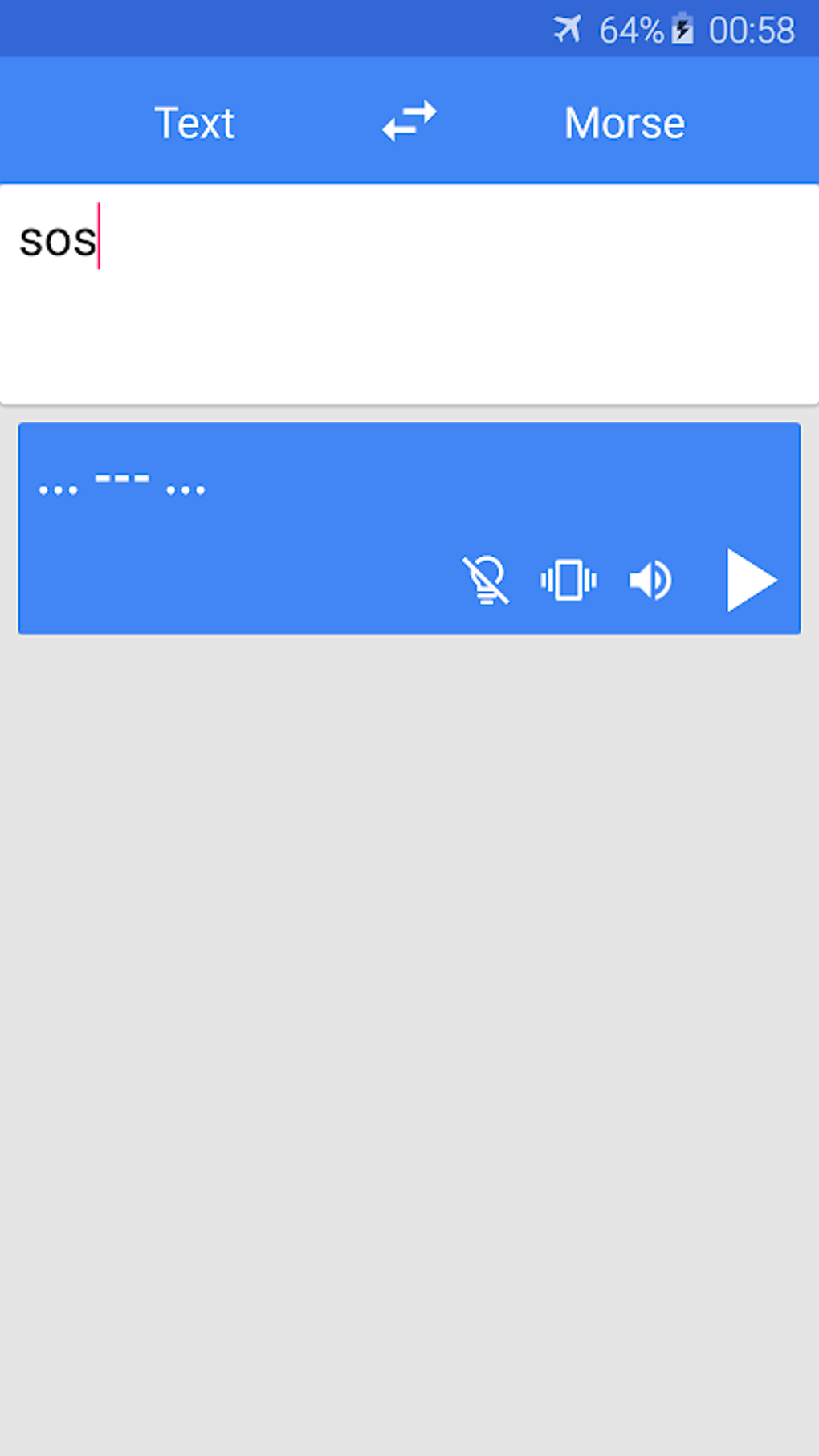The mobile screen capture illustrates a user interface in airplane mode with a 64% battery life, shown on the top status bar. The time is displayed as 00:58. Below the status bar, there is a top menu featuring various options, including text with two arrows pointing in opposite directions, indicating Morse code translation functionality.

The interface converts the typed message "SOS" into Morse code, displayed in a blue box with white text. Various icons are present, including a crossed-out light bulb, a rectangular shape with lines along its sides, a speaker icon with sound waves, and a play button, likely for audio playback of the Morse code message.

The background of the interface is gray, while the primary text area is white with black text. All accent text and icons on the blue sections are white, contrasting against a medium blue hue. Overall, the screen has a simplistic design with minimal additional elements.